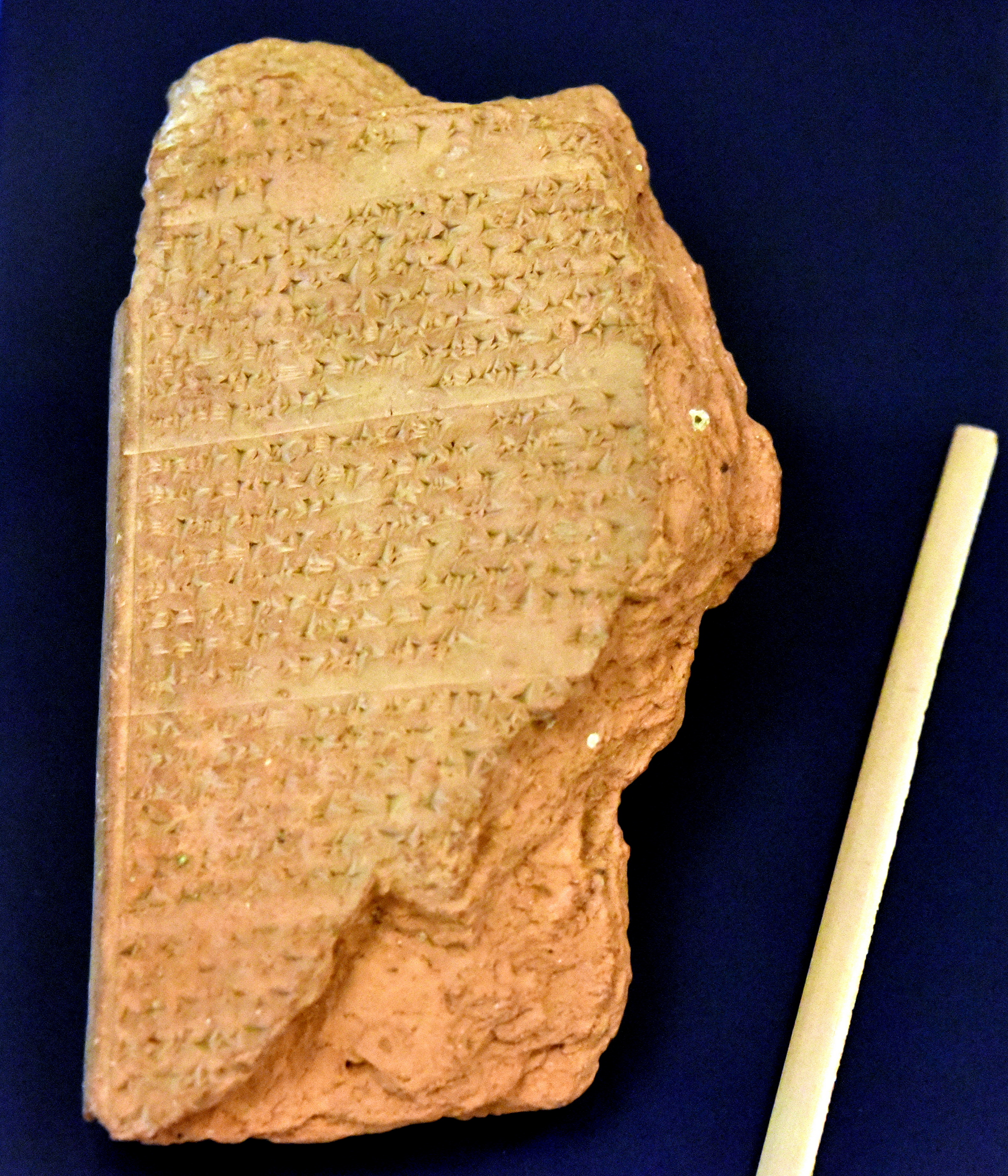The image showcases a large, irregularly shaped stone or rock with a peach or light brown color. The rock has a smooth left side and a jagged, chipped right side, giving it a somewhat rectangular but not quite geometrical shape. The surface of the rock has several speckles, adding texture to its appearance. Positioned next to the rock on the bottom right side of the image is a thin, tan rod that resembles a light yellow-colored cylinder or straw. The background is a plain navy blue, providing a stark contrast to the earthy tones of the stone and rod.